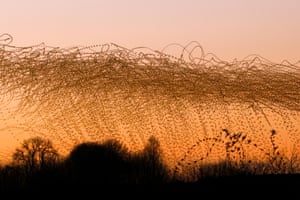In this outdoor color photo, the foreground is dominated by an intricate and tangled mass of netting or wiring, consisting of several hundred bunched-up strands. This chaotic mesh creates an almost interpretive art feel, composed of squiggly lines reminiscent of frantic scratches or scribbles. This jumble is set against a background that suggests the photo was taken around dusk or early sunrise, as the sky transitions from a deep and muted orange at the horizon to a grayish pink higher up. This serene and atmospheric backdrop is sparsely detailed, with vague silhouettes of trees and foliage hinting at an expansive natural setting. The bottom of the image introduces a dark, shadowy area, possibly indicative of a tree line or dense brush, adding to the mysterious and interpretive essence of the photo.